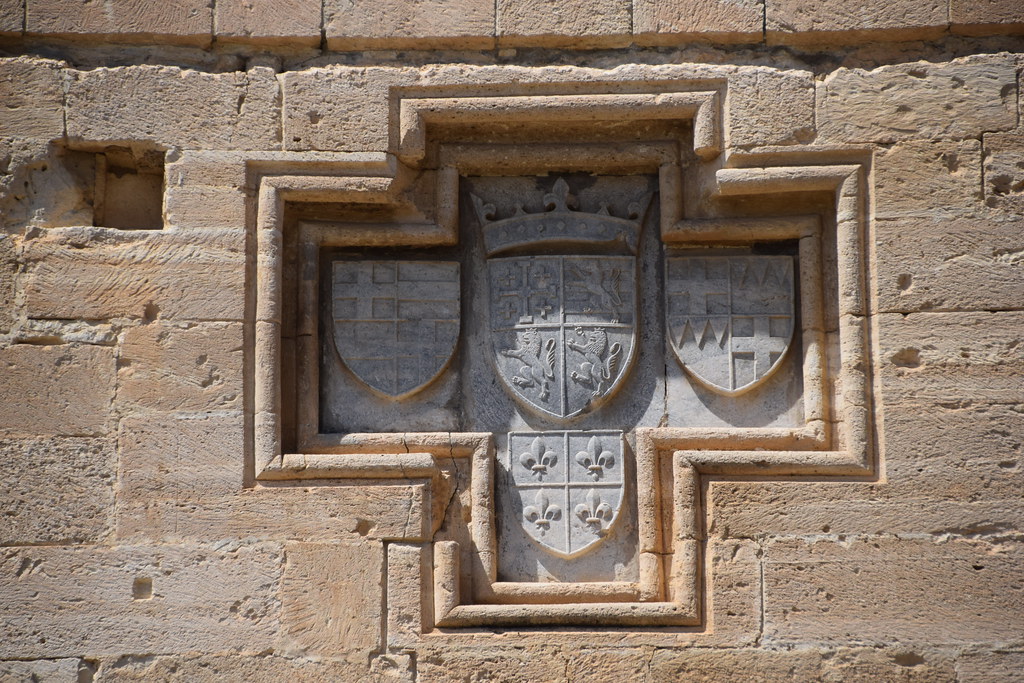The photograph captures a sand-colored brick wall composed of large, straight-cut stones meticulously arranged in straight lines. A single stone is missing on the upper left-hand side. Embedded within this wall is an intricately designed, indented cross. This central cross, appearing aged and possibly made of gray stone, features a crown at its pinnacle. Surrounding this crown is a prominent central shield divided into four quadrants; the upper left section displays a large cross flanked by smaller crosses, while the remaining sections are adorned with lion or griffin figures. Flanking the central shield are two smaller shields on either side, both split into four parts—these feature cross designs and triangular banners. At the base of the cross lies another shield segmented by fleur-de-lis designs. The entire relief is encased within a rounded stone border, accentuating its historical and aged appearance.